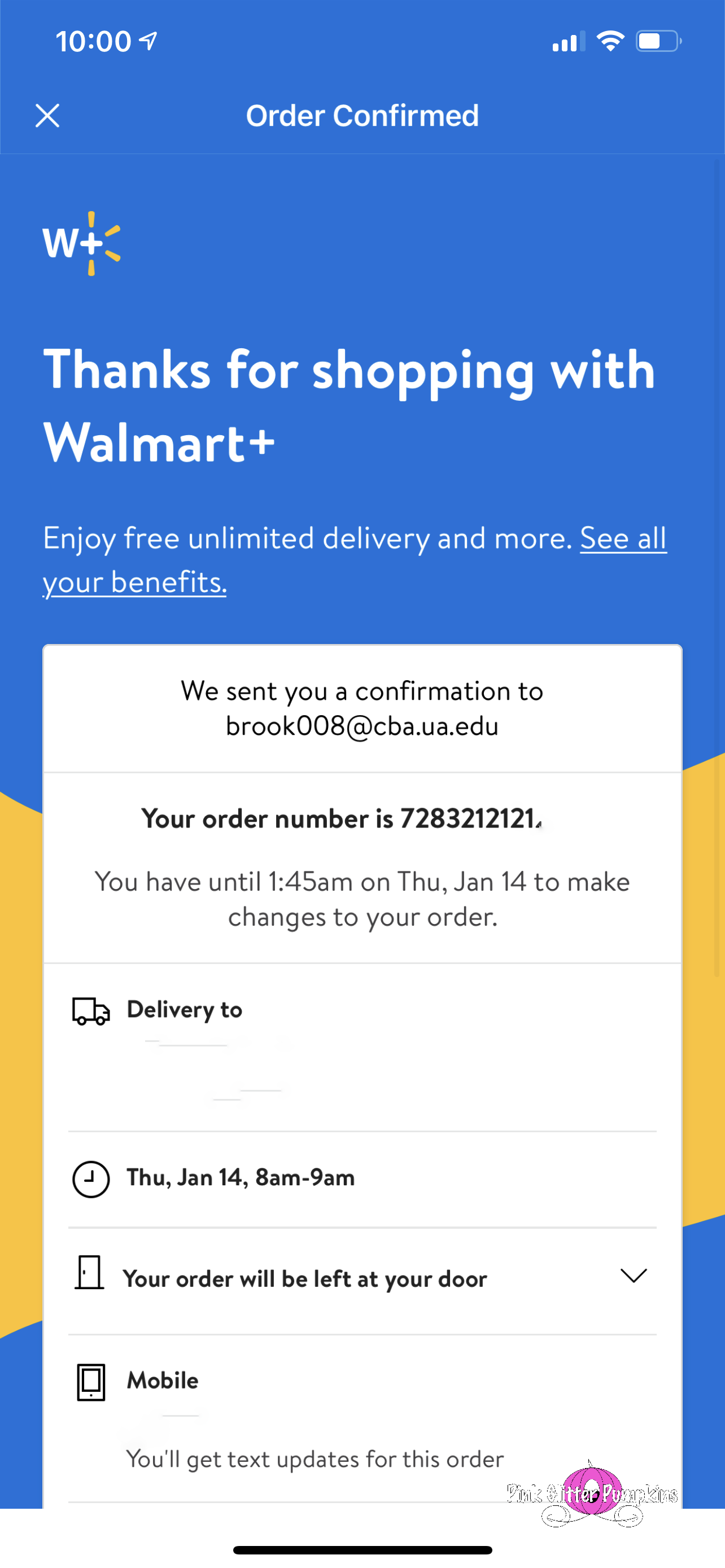The image displays a Walmart order confirmation screen with a light blue background. It is 10 o'clock, as indicated by the time display, and the battery icon shows it is halfway charged with a strong connection signal. At the top, the screen prominently states "Order Confirmed" accompanied by the Walmart logo. Below this, a message reads: "Thanks for shopping with Walmart Plus. Enjoy free unlimited delivery and more. See all your benefits," with an actionable link to view the benefits.

A white box dominates the center of the screen, stating, "We sent you a confirmation to brook008@cba.ua.edu." The order number is also provided, though redacted here for privacy. The message informs the user that they have until 1:45 PM on Thursday, January 14th to make changes to the order. The delivery details are outlined in a boxed section, specifying that the delivery will occur on Thursday, January 14th, between 8 a.m. and 9 a.m., and the order will be left at the door. A dropdown menu offers additional options under the delivery instructions.

At the bottom of this white section, an icon of a phone next to the word "Mobile" indicates that text updates will be sent for this order. To the right, there is a round, pink image with an indiscernible white element inside, adding a touch of color to the otherwise text-focused layout.